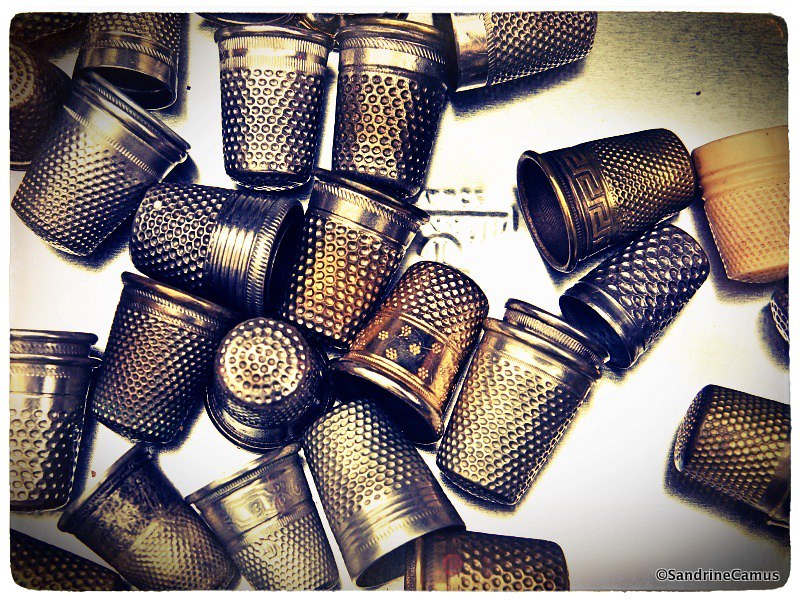A sepia-toned photograph showcases an intriguing collection of approximately 20 thimbles scattered across a white table, each featuring distinct designs and subtle variations. Most of the thimbles are chrome or silver metal, displaying the characteristic indents along their edges, though some carry warmer tones such as a unique tannish one on the right and a slightly purple-hued metal one. Among the metallic thimbles is a single rubber one, standing out from the lot. The thimbles lie in various orientations, with one notably positioned upside down. In the bottom right corner, the name "Sandrine Camus" is inscribed, potentially indicating the artist or owner of these thimbles. The sepia tone adds a vintage aesthetic to the overall scene.